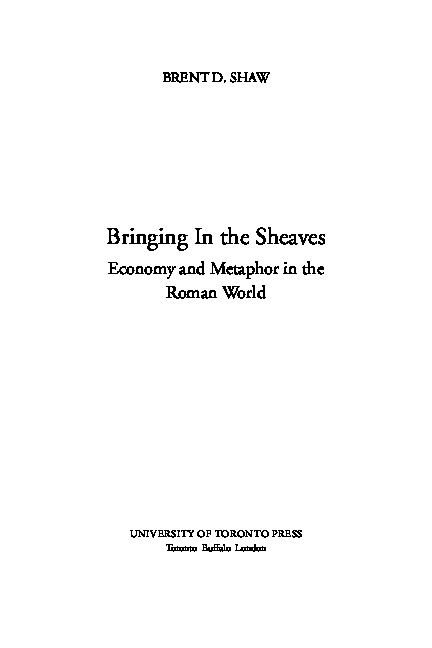This image is the interior cover page of a book with a clean, white background. The sophisticated serif font in black text contributes to an elegant and classic feel. Across the top, in a spacious layout, it reads "Brent D. Shaw." Below this, in three distinct lines, is the title "Bringing in the Sheaves," followed by the subtitle "Economy and Metaphor in the Roman World." Further down the page, again with ample spacing, it says "University of Toronto Press." Beneath this, in smaller text, it reads "Toronto Buffalo" with a final word that is too compressed to make out. The minimalist design and structured text give the page a deceptively simple and refined appearance.